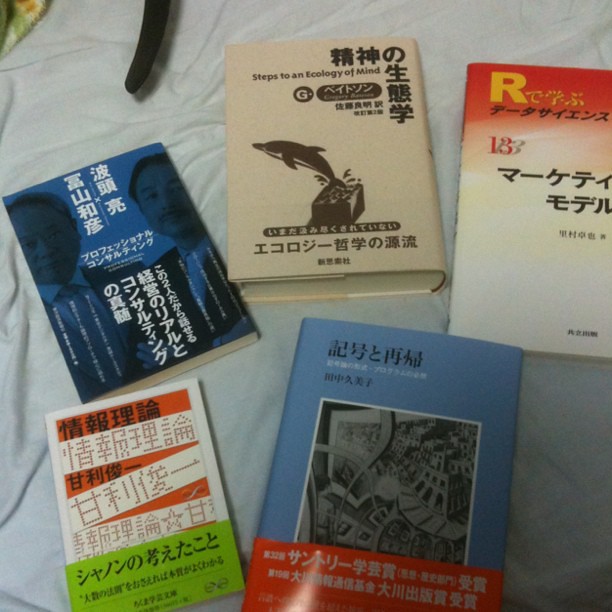The photograph presents five books laid out on a crumpled white fabric surface, resembling a bedspread or tablecloth. The composition features several colorful details: a touch of green, cream, and pinkish fabric in the upper left corner, and a small black cylindrical object nearby, which remains unidentified.

The books exhibit a variety of colors and designs, all featuring some form of East Asian writing, likely Chinese or Japanese. Arranged like a fan with three on the top row and two on the bottom, the books each bring their own distinctive features to the scene. The top left book is blue, adorned with images of two men, contrasting with a blue monochrome effect and white script. Adjacent to it is a light beige or tan book, presenting an image of a dolphin and the English title, "Steps to an Ecology of Mind." The third book in the top row transitions from red at the top to white at the bottom, topped with a prominent yellow letter 'R.'

Moving to the bottom row, the fourth book exhibits a visually striking red and white striped pattern accompanied by a green band, all containing more of the characteristic script. The final book on the bottom right is blue, featuring a central black-and-white picture, though the exact image remains unclear, and a red band across the bottom with additional text.

This richly detailed scene captures the interplay of vibrant colors, varying textures, and intriguing designs, all centered around the enigmatic and culturally rich eastern texts.